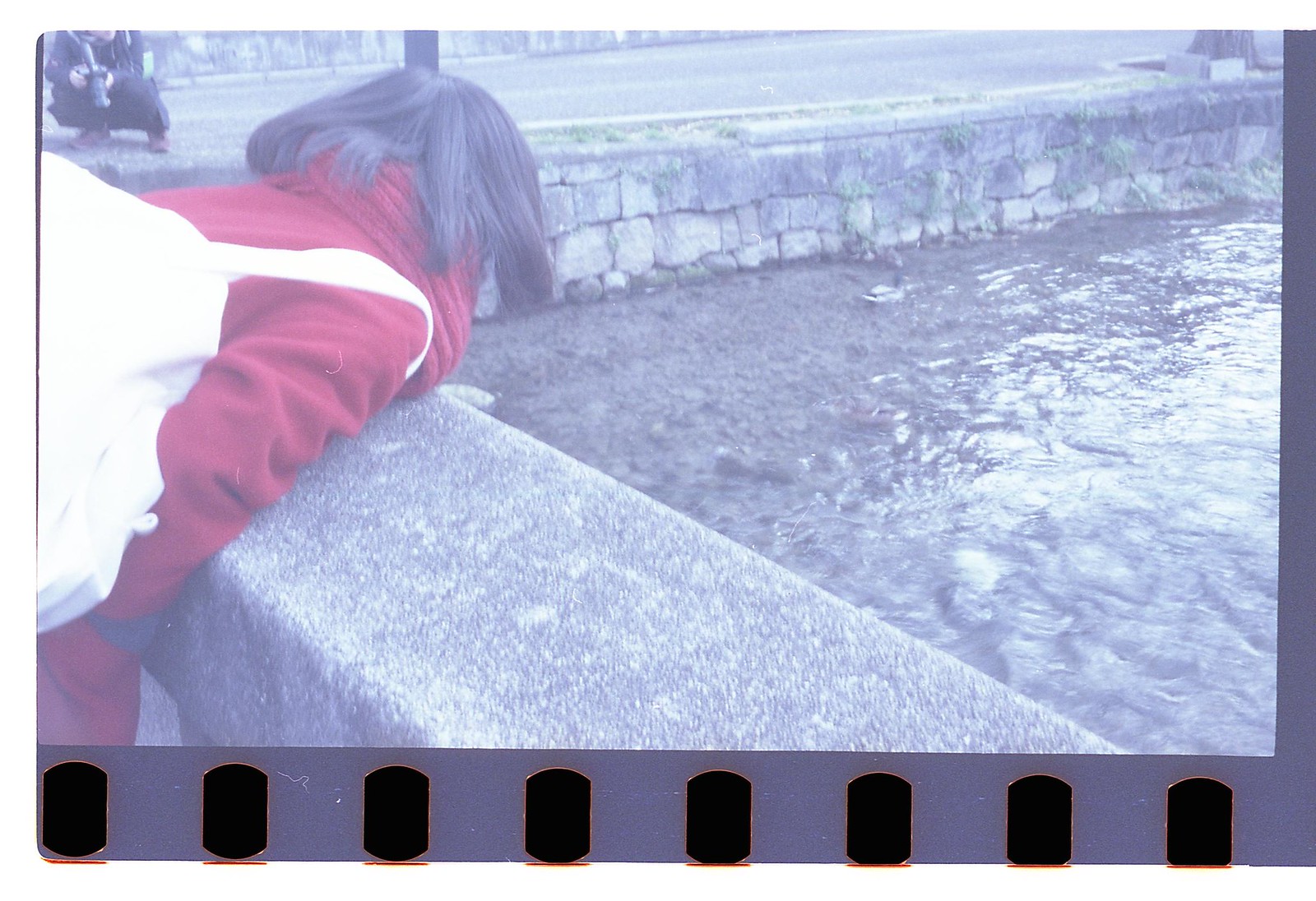In this overexposed, landscape-oriented photograph, a scene of muted light colors is depicted. A concrete wall, which extends diagonally from the bottom right toward the upper left corner, dominates the foreground. A woman with dark, shoulder-length hair and clad in a red coat and scarf leans over this wall. She carries a white bag over her right shoulder, and her gaze is directed toward the gray, rippled water below. In the background, beyond this wall, there's a stone guardrail running left to right, indicating the river’s encasement in concrete or stone for stability. Another person, visible in the upper left corner, squats at the river's edge, holding a camera and peering into the water. The image has a dark gray border with holes reminiscent of old film negatives, adding a vintage feel to the photograph. Overall, it seems to be a chilly day, as suggested by the woman's attire and the general ambiance of the image.